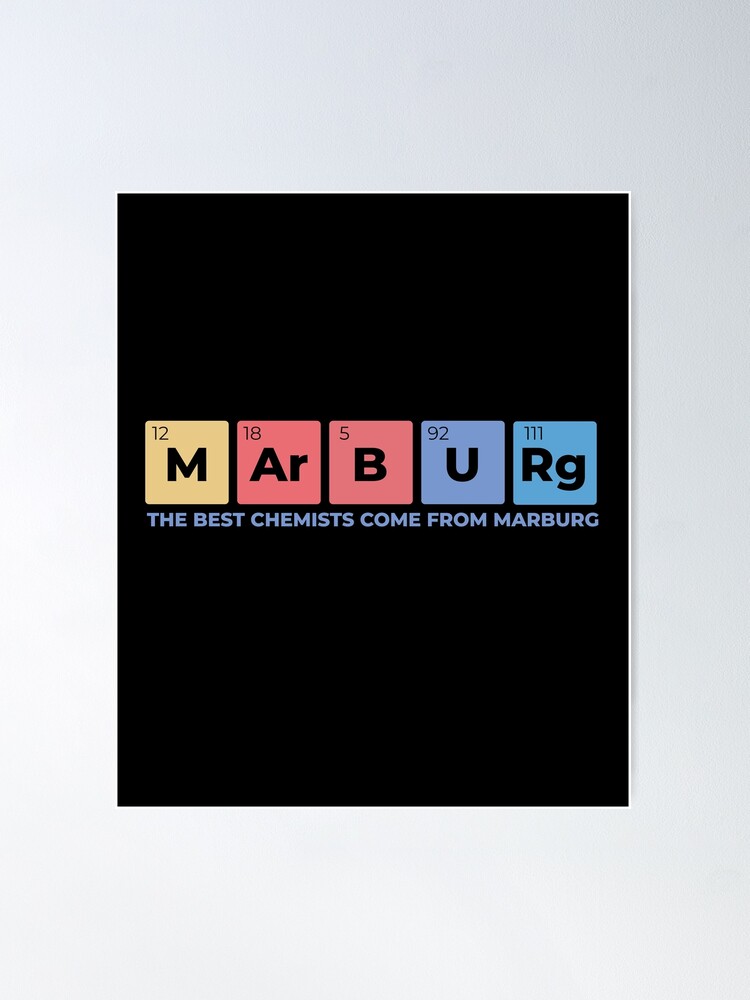The image is a promotional infographic set against a black background, centrally featuring a series of periodic table tiles that spell out "MARBURG." Each tile has a different background color and atomic number. The sequence begins with a light blue tile for element 12 (M), followed by a yellow tile, and then two pink tiles: one for element 18 (AR) and one for element 5 (B). Next is a light blue tile for element 92 (U), and it concludes with a vibrant sky blue tile for element 111 (RG). Beneath these tiles, in all-caps light blue font, is the text "THE BEST CHEMISTS COME FROM MARBURG." Both the tiles and text are centrally aligned on the black background, giving the image a clean and focused appearance.